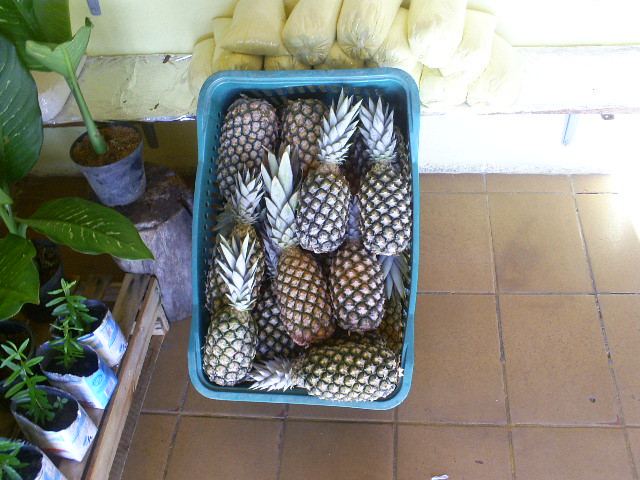In this photograph, there is a detailed scene featuring a blue laundry basket brimming with pineapples. The basket is positioned on its side, revealing numerous pineapples inside, characterized by their grayish-yellow hues with light, almost white-green, spiky leaves. The setting appears to be a light brown tiled floor with small square tiles. Behind the basket are several bags, which seem to contain a yellow substance, possibly cooking ingredients. 

To the left of the basket, there is a variety of potted plants. Prominently, a dark-colored pot holds a larger green leafy plant. Surrounding this pot, several smaller containers, which look like cut-down planters, contain dirt and small green sprouts. Further in the background, atop a wooden stump, another black pot with dirt holds a tall green plant with lush foliage. Additionally, a wooden crate or pallet is visible, with four paper envelopes filled with dirt and sprouting green leafy growths standing upright on top of it.

The setting is framed by a white cement wall, partially covered with a tinfoil-lined shelf, where several baggies containing a light powdery substance are piled on top of one another. The overall composition offers a vivid and intricate glimpse into an organized yet natural arrangement of objects and plants.